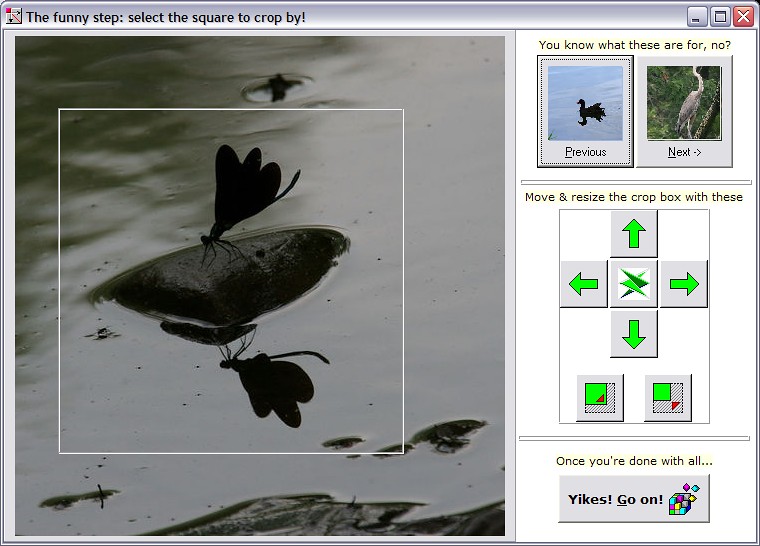The screenshot depicts an interface from a photo-editing computer program with a light silvery-blue border. At the top, the interface features a header in black print on a white and blue background that reads, "The funny step: Select the square to crop by!" Below this header, dominating the left side of the image, is a macro photograph of a dark, winged insect, possibly resembling a butterfly or black bug, perched on what appears to be a black rock or perhaps the head of a small mammal, such as a manatee, in dark water. This photograph is bordered by a gray crop box.

To the right of the main photograph, the interface displays two smaller images stacked vertically: the upper image is that of a blue duck in water labeled "previous," and the lower image features a gray crane with a long white neck against a green background, labeled "next." Above these images is a small black print stating, "You know what these are for." Below these images, a section of green directional arrows—pointing up, down, left, and right—enable the user to move or resize the crop box.

Further down, there are smaller boxes likely indicating additional orientation options for the image. At the bottom of the interface, in a gray box, there's text that reads, "Once you're all done," followed by a blue box with the words "Yikes, go on," next to a cubic figure emitting smaller inverted squares. The primary focus remains the dark-winged insect on the rock in the water, as integrated into this intricate editing tool interface.